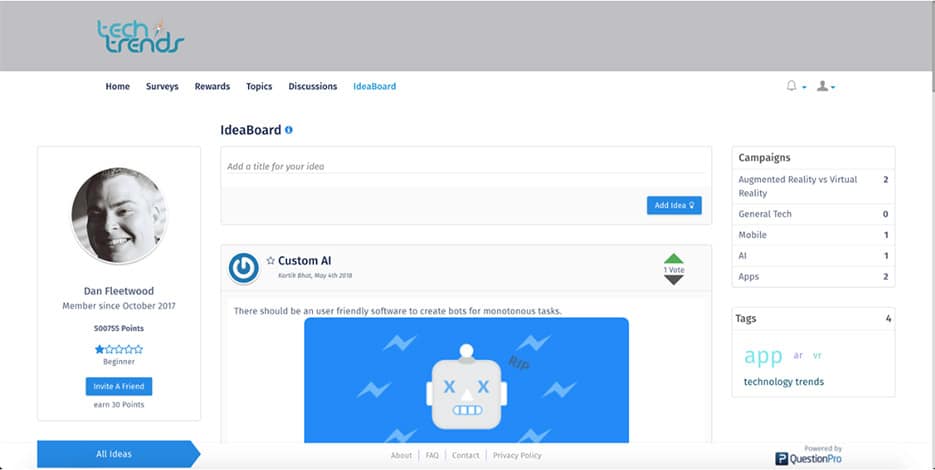In this image, we see a screenshot of a web platform called TechTrends, which resembles Twitter and appears to be displayed on a desktop due to its widescreen layout. At the top, beneath the TechTrends logo, there is a navigation bar with links labeled Home, Surveys, Rewards, Topics, Discussions, and Idea Board. The current page displayed is the Idea Board, which is focused on adding and sharing ideas.

Just below the Idea Board heading, there is a text box for users to enter the title of their idea, accompanied by a blue "Add Idea" button on the bottom right of the box. This setup suggests users can easily submit their ideas by typing them out and clicking the button.

An example of an idea is already present below the text box, titled "Custom AI." The accompanying description reads, "There should be a user-friendly software to create bots for monotonous tasks." This indicates that a user has proposed a concept that aims to streamline repetitive tasks through automation.

To the right of the idea, there are upward and downward arrows, allowing users to vote on the idea positively or negatively. 

On the left side of the screen, there is a member profile section displaying the name "Dan Fleetwood" along with a picture of his face, suggesting he might be the user who submitted the idea or is otherwise significant on the platform.